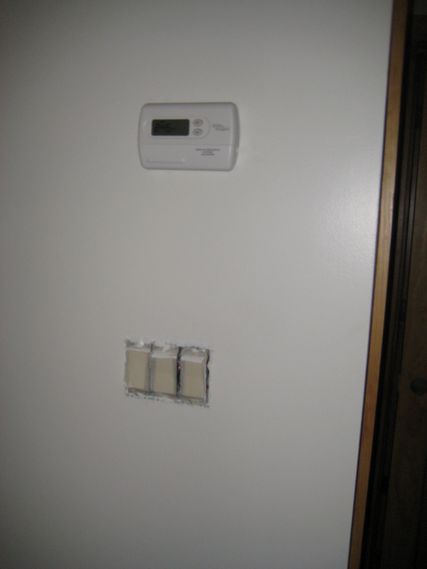The image captures a close-up of what appears to be the side panel of a white cupboard or wall. The surface is uniformly white, except for the right edge, which has a brownish tint. Near the bottom center of the panel, there is a noticeable square area with discoloration that could either be a hole or a framed picture. This area features three light brown vertical bars, each topped with white dots, arranged side by side. Toward the top of the panel, there is a small, four-cornered square piece affixed to the wall. This piece has small writings on both the top and bottom right corners. Additionally, it includes two circular buttons aligned vertically, one above the other. The square piece also contains a small screen with a green background, displaying numbers in black.